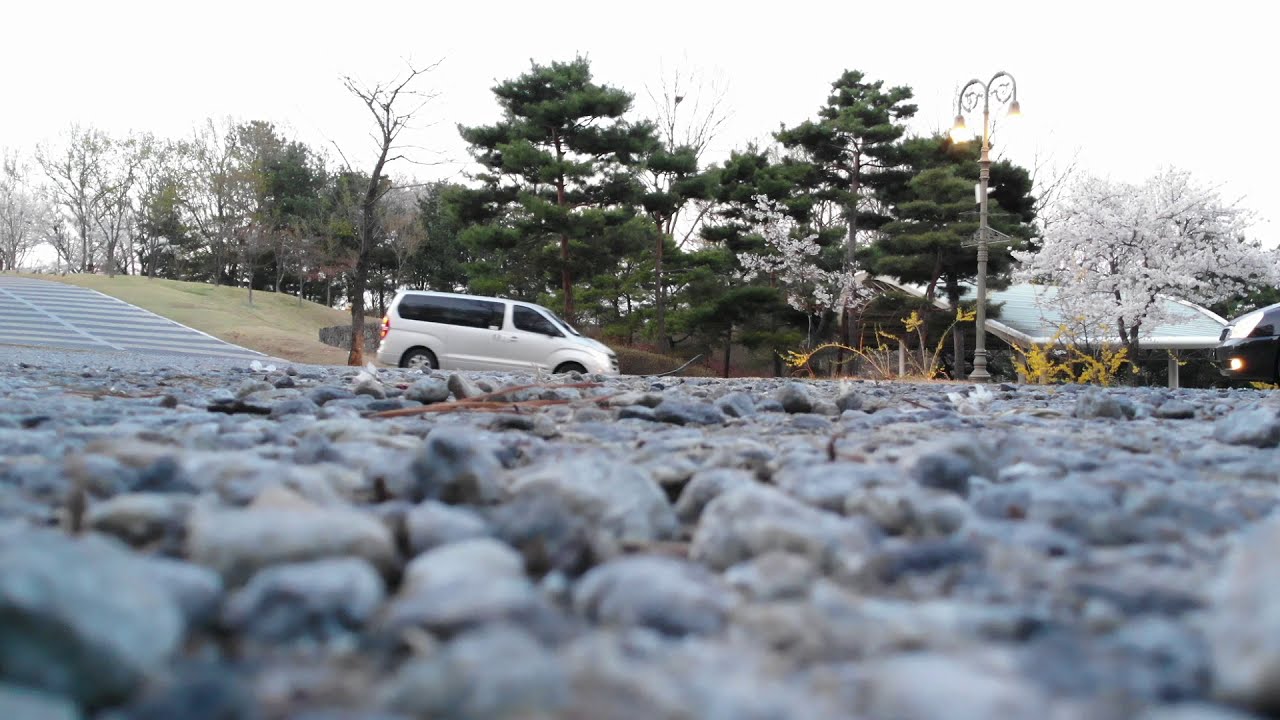A color photograph in landscape orientation captures a rugged, rocky field or parking lot from a ground-level vantage point. In the mid-ground, slightly to the left of center, a beige passenger van can be seen driving along a street. The left side of the image features a grass-covered slope with concrete steps descending it. In the background, tall, dark green trees line the scene, providing a natural border. To the right, a dark-colored house with a snow-covered roof peeks out from behind an elegant lamppost with twin curved lanterns. The composition evokes a serene suburban environment, possibly a state park or residential area, with a touch of architectural charm added by the lamppost and gazebo with lights visible in the same direction.